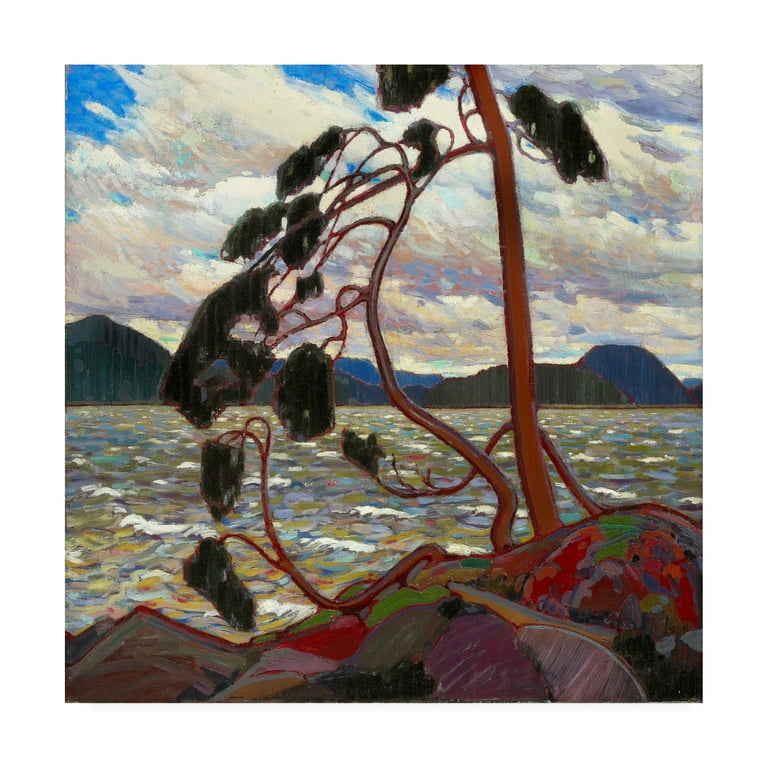The painting, measuring approximately four to five inches square, depicts a striking tree growing from a vividly colorful rock at the edge of a cliff overlooking a dynamic ocean. The rock, steeped in hues of green, red, purple, orange, yellow, and blue, appears as if splashed with paint, creating a captivating mosaic of colors. From this rock emerge three thin brown trunks, each with a unique form: one rises straight up, the second bends into an S-shape, and the third dips down before curving upward again. These trunks are adorned with about 10 green leaves scattered along their lengths. The ocean below is rendered in shades of green, blue, and purple, with white-capped waves adding texture to the scene. Beyond the ocean, a series of blue and green mountains provides a serene backdrop, topped with thick white clouds tinged with oranges and yellows, with glimpses of dark blue sky peeking through.